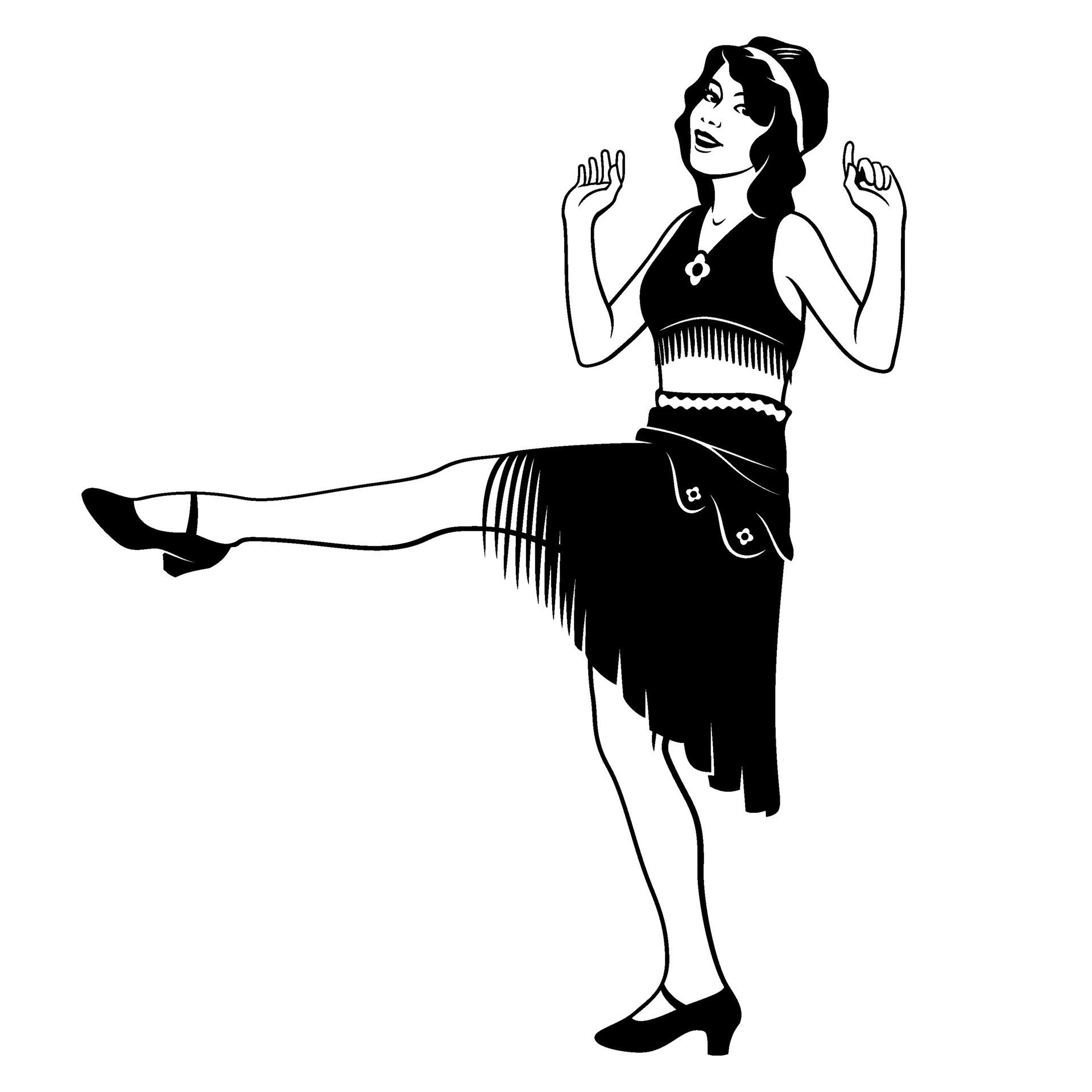This detailed black-and-white illustration depicts a woman in mid-dance, reminiscent of a flapper from the 1920s. She stands against a plain white background, her right leg kicked up to the left at a right angle, while her left foot remains grounded. Her arms are raised to about ear level, adding a sense of dynamic motion. She has long black hair adorned with a white headband and wears a dark black dress that features a white section around the waist and frills at the bottom. The dress has a low-rise top, exposing a bit of her midriff. She also sports a flower brooch near her neckline and black high heels. Her head is slightly tilted up as she looks towards the center of the image, making a spirited facial expression. This comical and stylized depiction captures the vibrant energy of a dancer lost in her own world.